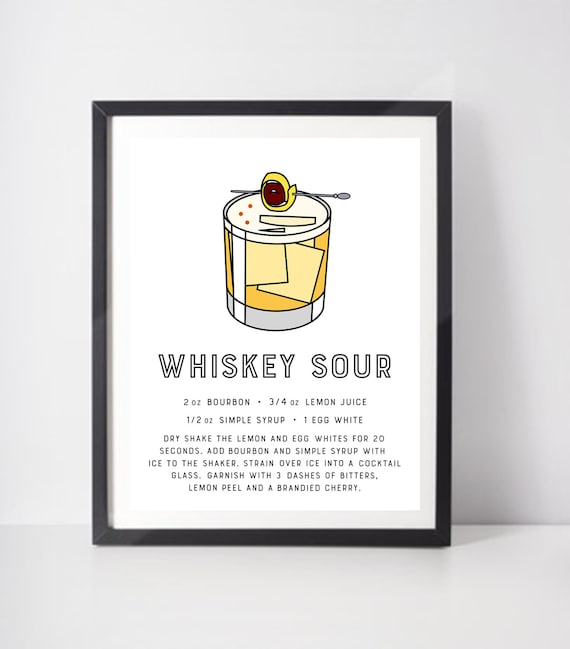Displayed against a white background is a striking framed panel featuring a detailed recipe for a whiskey sour. The black frame is accentuated by a light gray outline, adding depth to the composition. Inside, on a pristine white surface, there is a stylized drawing at the top: a skewer piercing a round object, resembling an olive or cherry, positioned above a glass filled with an orange-colored liquid and ice cubes. 

The text is presented in clear, black capital letters, reading "WHISKEY SOUR," followed by the specific measurements: "2 ounces bourbon, 3/4 ounce lemon juice, 1/2 ounce simple syrup, 1 egg white." Further instructions are meticulously listed: "Dry shake the lemon and egg whites for 20 seconds. Add bourbon and simple syrup with ice to the shaker. Strain over ice into a cocktail glass. Garnish with three dashes of bitters, lemon peel, and a brandied cherry." This visually engaging frame effectively conveys the classic cocktail recipe with both precision and aesthetic appeal.